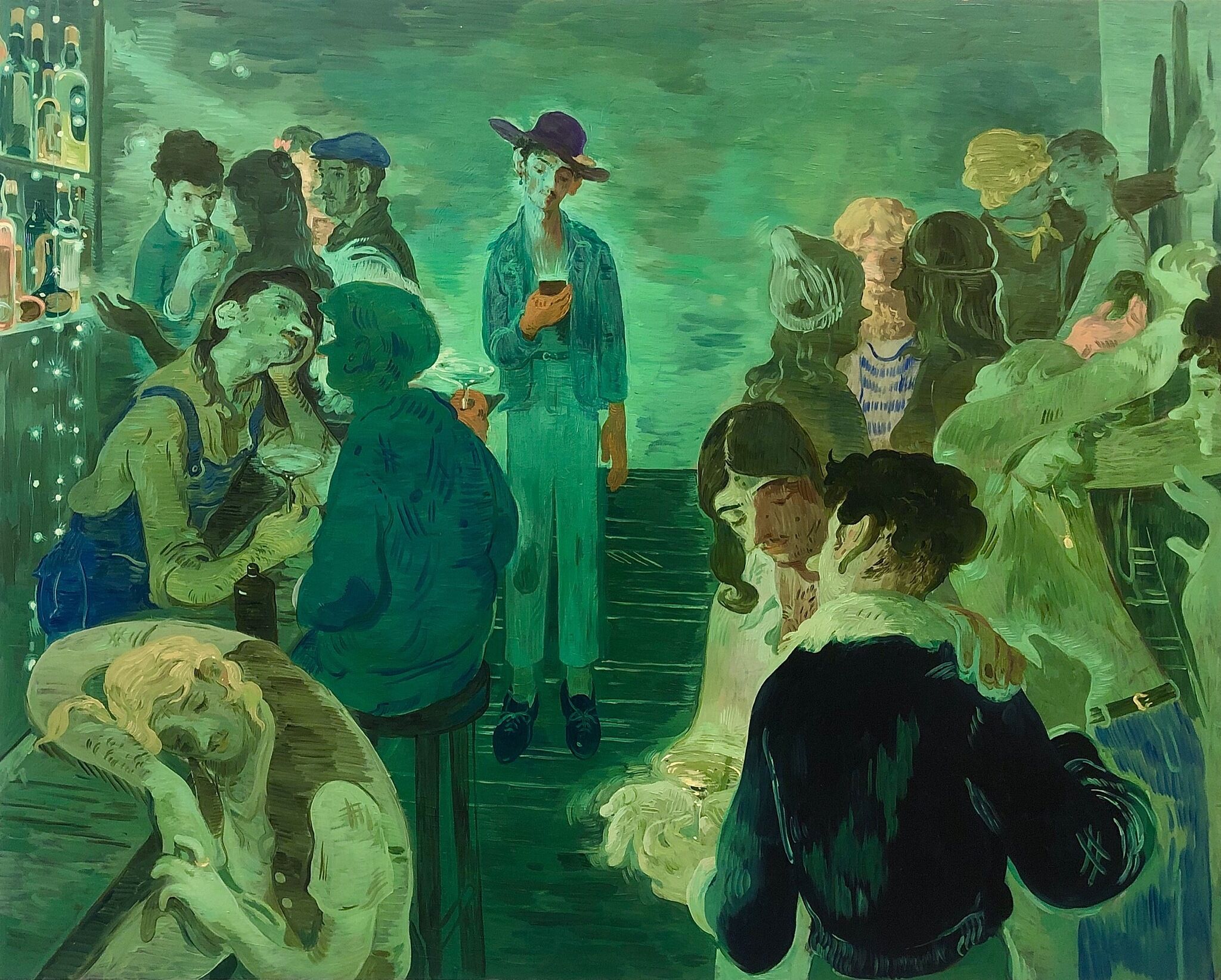This impressionistic painting captures a vibrant bar scene set against a dark green and blue color palette. The focal point is a man in the center, dressed in greenish pants and a blue jean jacket, holding a dark beer in his hand, and wearing a broad, dark blue hat. Surrounding him, the floor and walls are a dark green, blending with the background strokes of horizontal gray and green that suggest a lively but subdued atmosphere. 

On the left side of the painting, a busy bar area features a bartender tending to shelves lined with alcohol bottles. Some patrons are seated at tables or benches, with one man resting his arm on the counter as if he's dozing off. The right side is animated with dancers in dark jackets and white blouses, some engaging in close embraces that suggest they might kiss. Among them, a person in brown clothes stands out, and another figure is seen carrying a champagne glass. The overall scene is a blend of leisure and intimacy, rendered in rich green and blue tones that envelop the entire bar environment.